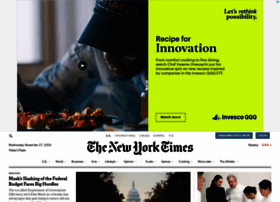This image features a screenshot from The New York Times website. The central focus is a Wordle game displayed on a smartphone screen, prominently showing the distinctive color-coded feedback—gray, green, yellow, and black squares—that represent the game's hints. The smartphone and Wordle game have a vivid green background, capturing immediate attention.

Below the Wordle game display, "The New York Times" is clearly written. The image also includes a series of thumbnail visuals and article previews. The first thumbnail shows what appears to be a scene of a highway, accompanied by three articles. Beneath that, there is an article highlighted by an image of a cabin nestled in a picturesque setting. Under this, a smaller article is noted, followed by two additional thumbnail images below it, adding to the layout's rich and varied content presentation.